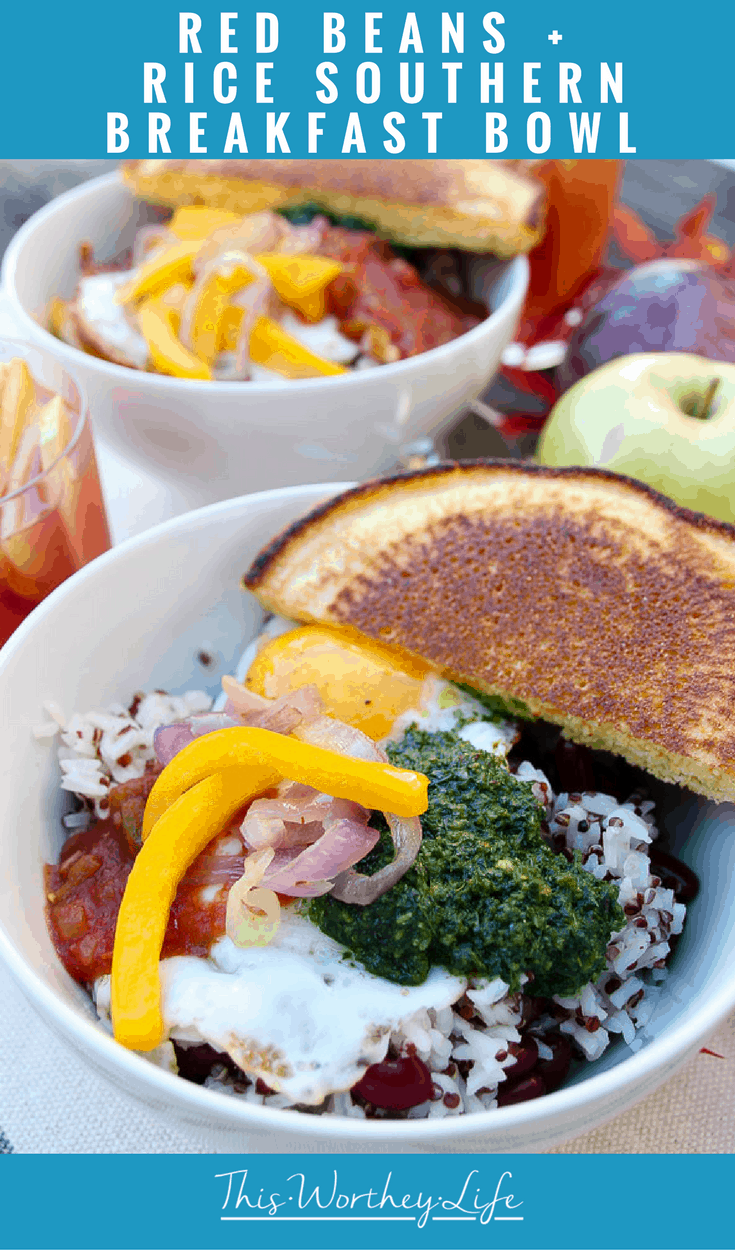This image is an advertisement for a restaurant or food service, prominently featuring a "Red Beans plus Rice Southern Breakfast Bowl." The composition includes a blue banner at the top and bottom; the top banner has white text that reads "Red Beans plus Rice Southern Breakfast Bowl," while the bottom banner has elegant white cursive text stating "This Worthy Life."

Centrally, the photograph showcases two white porcelain bowls placed on a canvas burlap-like placemat. Both bowls appear to contain similar contents: a hearty mixture of rice with various black seeds, a green plant-like puree, and bread. In one bowl, there's also half a pancake, a sunnyside egg, black beans, collard greens, sautéed onions, yellow bell peppers, and possibly pickled onions and salsa.

Accompanying the bowls are a green and red apple situated between them and a clear glass filled with a brown liquid, likely lemon iced tea, on the left side of the image. The overall presentation is rustic and inviting, aiming to highlight the richness and variety of the Southern breakfast offered.